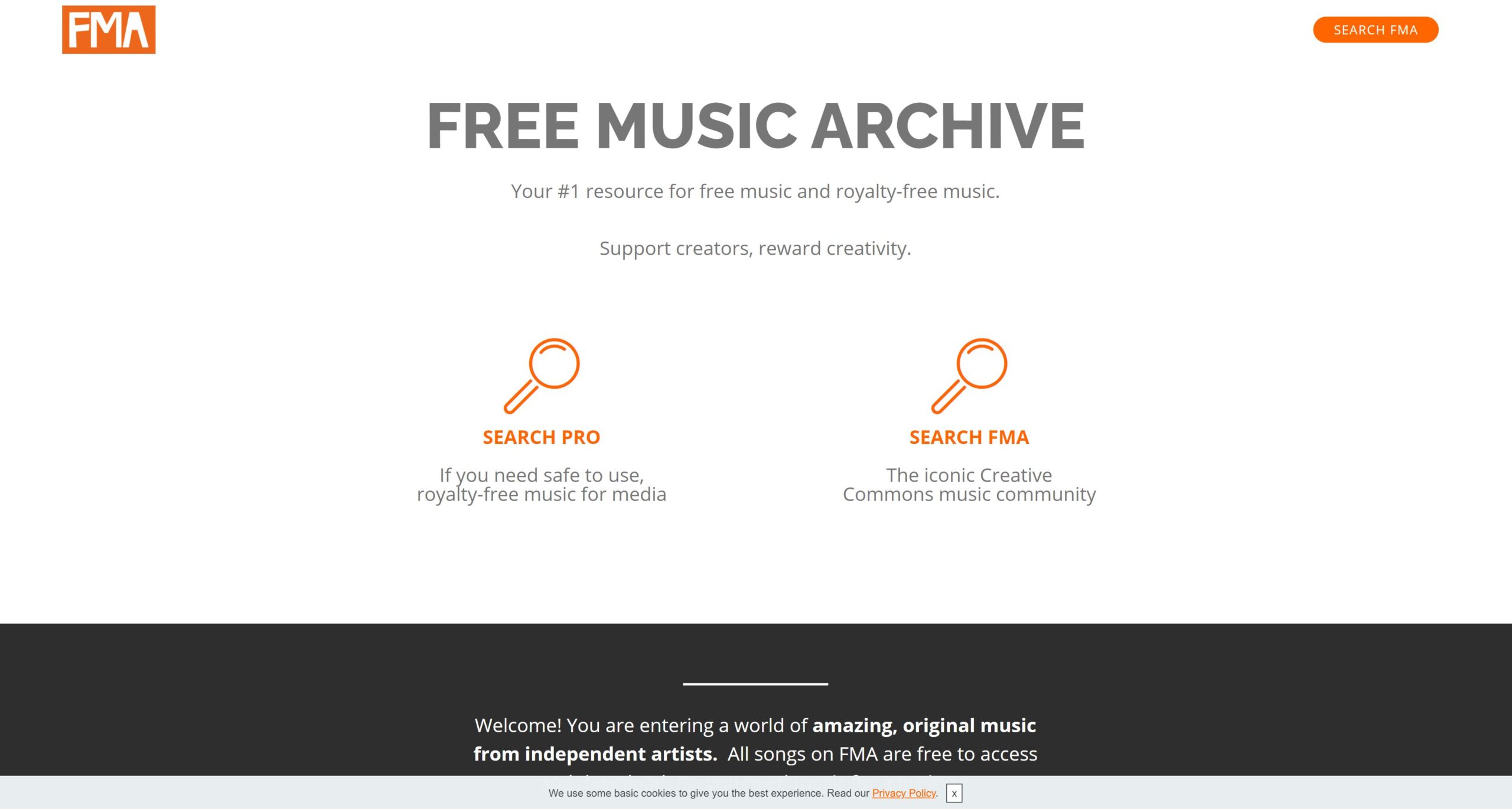This image features a webpage for the Free Music Archive (FMA). Dominating the center of the page is a clear white background, prominently displaying the text "Free Music Archive" in capital letters and light gray font. In the top left corner, an eye-catching orange rectangle with white lettering houses the acronym "FMA". On the top right, a small search button labeled "Search FMA" is visible.

At the very bottom of the page, a large black rectangular box catches the eye, with text that reads, "Welcome. You are entering a world of amazing original music from independent artists. All songs on FMA are free to access." 

In the center of the page, two search buttons are prominently highlighted, each adorned with magnifying glass icons. The left button, labeled "Search Pro," is for finding royalty-free music suitable for media use. The right button, labeled "Search FMA," notes underneath it, "the iconic Creative Commons music community.” This website serves as a robust search engine for discovering music on the Free Music Archive platform.